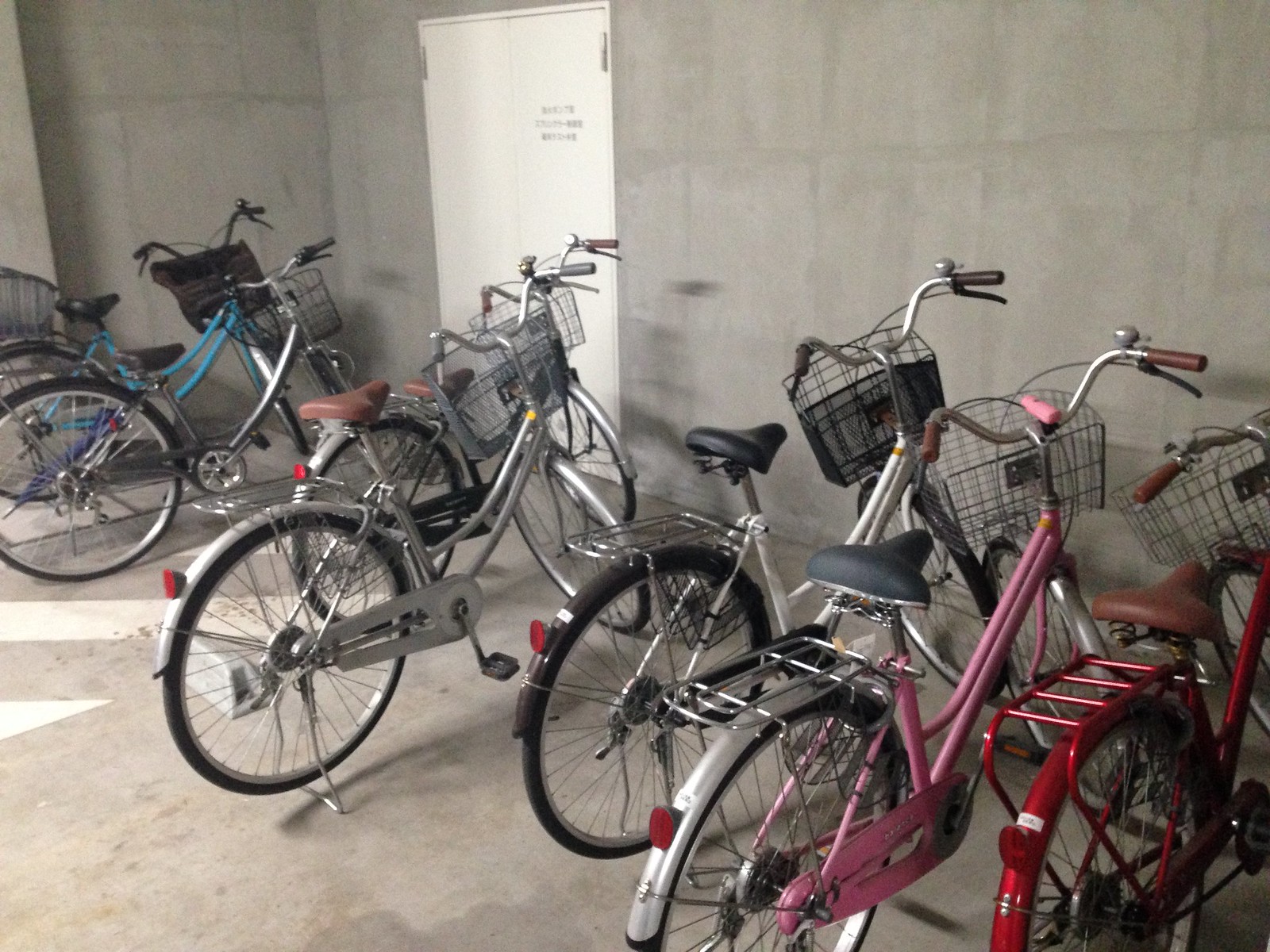This photograph features seven bicycles lined up side-by-side against a grey wall with a double white door that has a sign with unreadable black writing on it. The room has a grey floor. Starting from the right, the first bicycle has a red frame with a brown seat, brown handlebars, and a basket. The second bicycle from the right has a pink frame, a grey seat, brown handlebars, and a bell. Next to it is a bike with a light grey frame, a black seat, and black handlebars, also equipped with a basket and bell. The fourth in line is a light grey bike with a brown seat and light grey handlebars. Slightly obscured behind this is another bike with brown handlebars and a light grey frame. The sixth bicycle features a light grey frame, black seat, and black handlebars. Finally, the bicycle on the far left has a light blue frame, black seat, and black handlebars. All seven bicycles have front baskets for carrying items, and some also have rear carriers and stands propping them up.